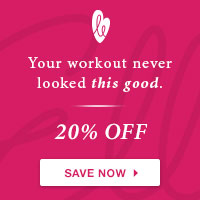**Caption:**
A small, square advertisement with a vibrant red background, featuring darker red swirls that create looping patterns. At the top center, there is a lopsided white heart adorned with red cursive lines resembling an intertwined 'L' and 'E'. Directly below the heart, white text reads: "Your workout never looked this good." The word 'Your' is the only one with a capitalized 'Y'. An ombre effect white line serves as a separator, below which the text "20% OFF" is prominently displayed in all caps. At the bottom of the ad, a white rectangular button with red uppercase text reads "SAVE NOW" and includes a small red arrow.